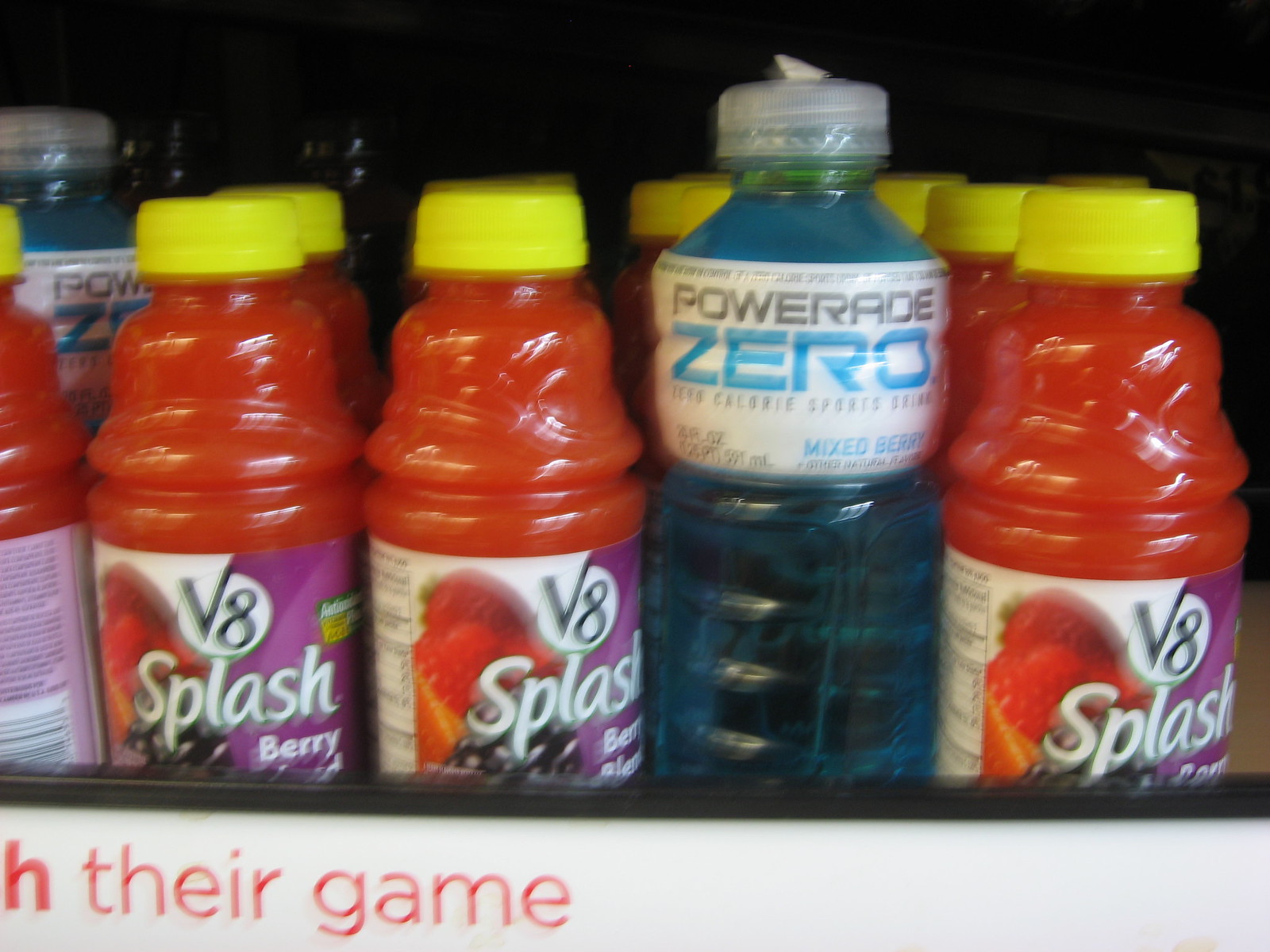A detailed photograph captures a store shelf packed with various beverage bottles. On the left, a row of Powerade Zero bottles stands upright, each containing a bright blue liquid labeled "Mixed Berry." Adjacent to them, several V8 Splash bottles with yellow caps are visible, filled with an orange-colored drink. The V8 Splash labels feature images of strawberries and purple berries. The background of the scene appears dark, indicating that the shelf might be inside a cooler. Above the neatly arranged bottles, the red letters "T-H-E-I-R game" stand out, adding a distinctive touch to the composition.